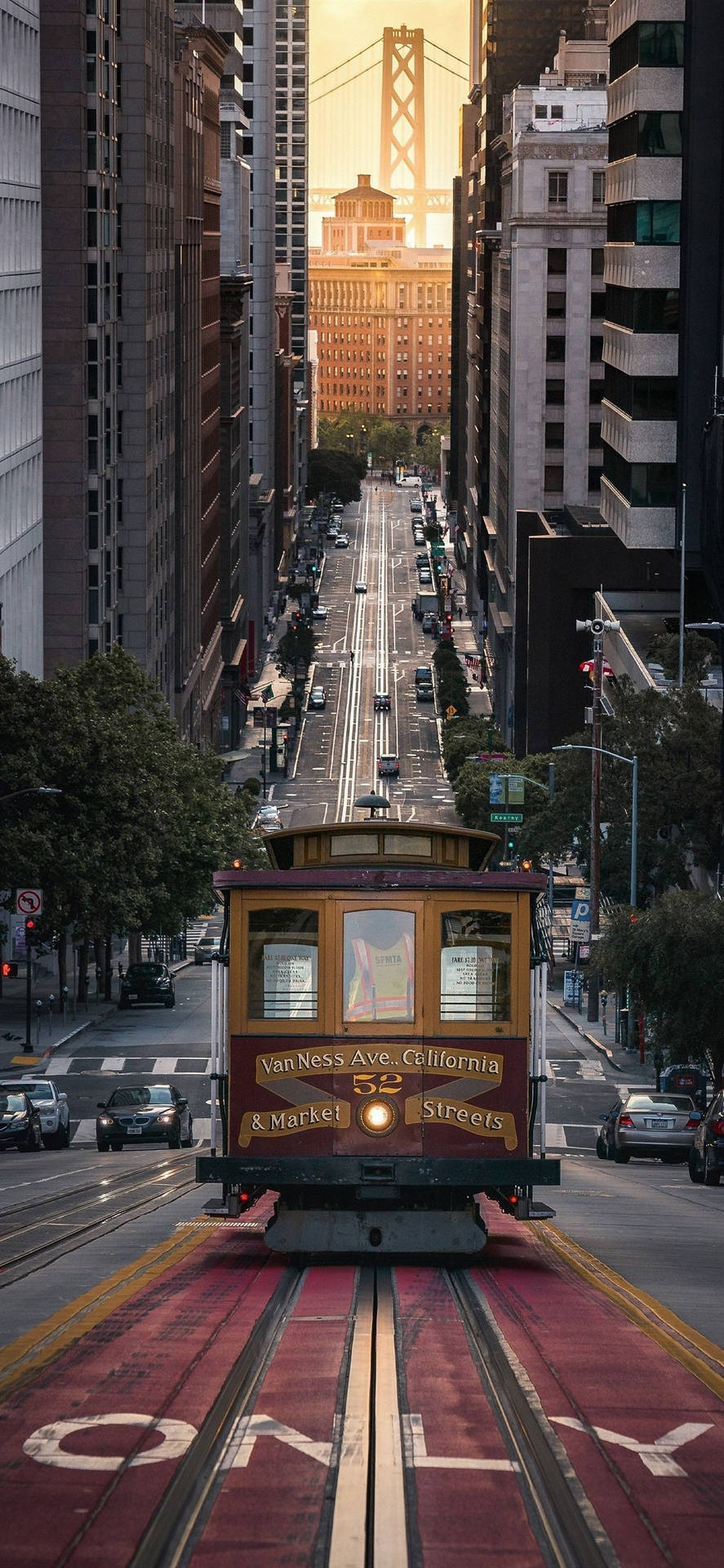This detailed photograph captures a quintessential San Francisco scene: a burgundy-colored trolley navigating the steep incline of Van Ness Avenue. The trolley bears the text “Van Ness Avenue, California” and “Market Street,” and it prominently displays the number 52 alongside the label “Endmarket Streets.” The trolley itself is painted in a rich Bordeaux-burgundy hue with bronze accents, complementing the similarly colored trolleyway. In the middle of the street, the trolley moves downhill, with an employee wearing a yellow or green safety vest inside. Surrounding the trolley are numerous cars moving in opposite directions, flanking the trolley's dedicated path. The steepness of Van Ness Avenue is highlighted by a noticeable slope change about one-fourth down the image. In the radiant distance, the iconic Golden Gate Bridge stands tall, partially obscured by a sunlit building. While the further background gleams brightly under the sun, the foreground, framed by towering buildings, appears gray and shadowed, emphasizing the contrasting atmospheres within the cityscape.